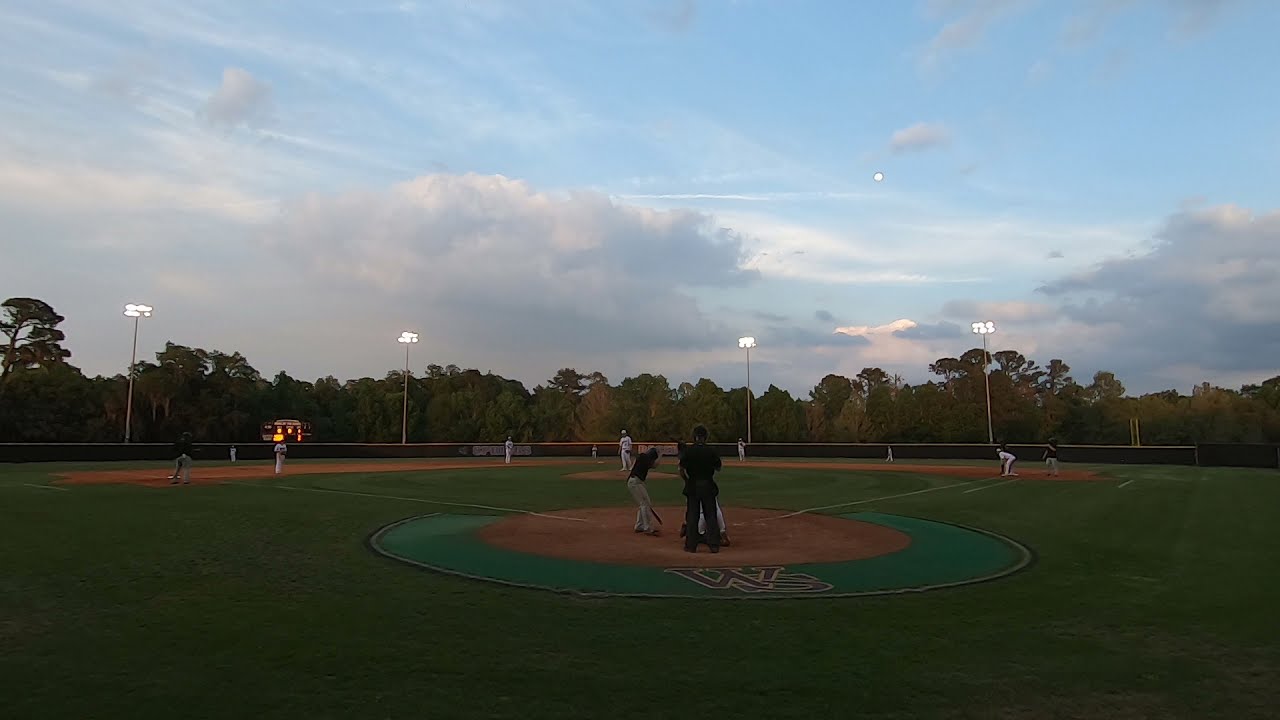At dusk, beneath a light blue sky adorned with white clouds, a lively baseball game unfolds on a field encircled by green trees at the horizon. The meticulously maintained field showcases verdant grass punctuated by brown dirt patches at the bases and batter's box, while the batter’s circle emblazoned with the letters "WS" stands out prominently. Stadium lights are already illuminated, casting a soft glow over the scene, enhancing the evening’s ambiance. In the midst of the game, a player clad in black is poised to catch the ball, while another, dressed in a gray and black ensemble, prepares to bat. Distant figures, hinting at their roles as pitcher and outfielders, blend into the background, their uniforms appearing gray or white under the encroaching twilight. The scene is a harmonious blend of greens, blues, and browns, capturing the tranquil yet anticipatory atmosphere of a baseball game at dusk.